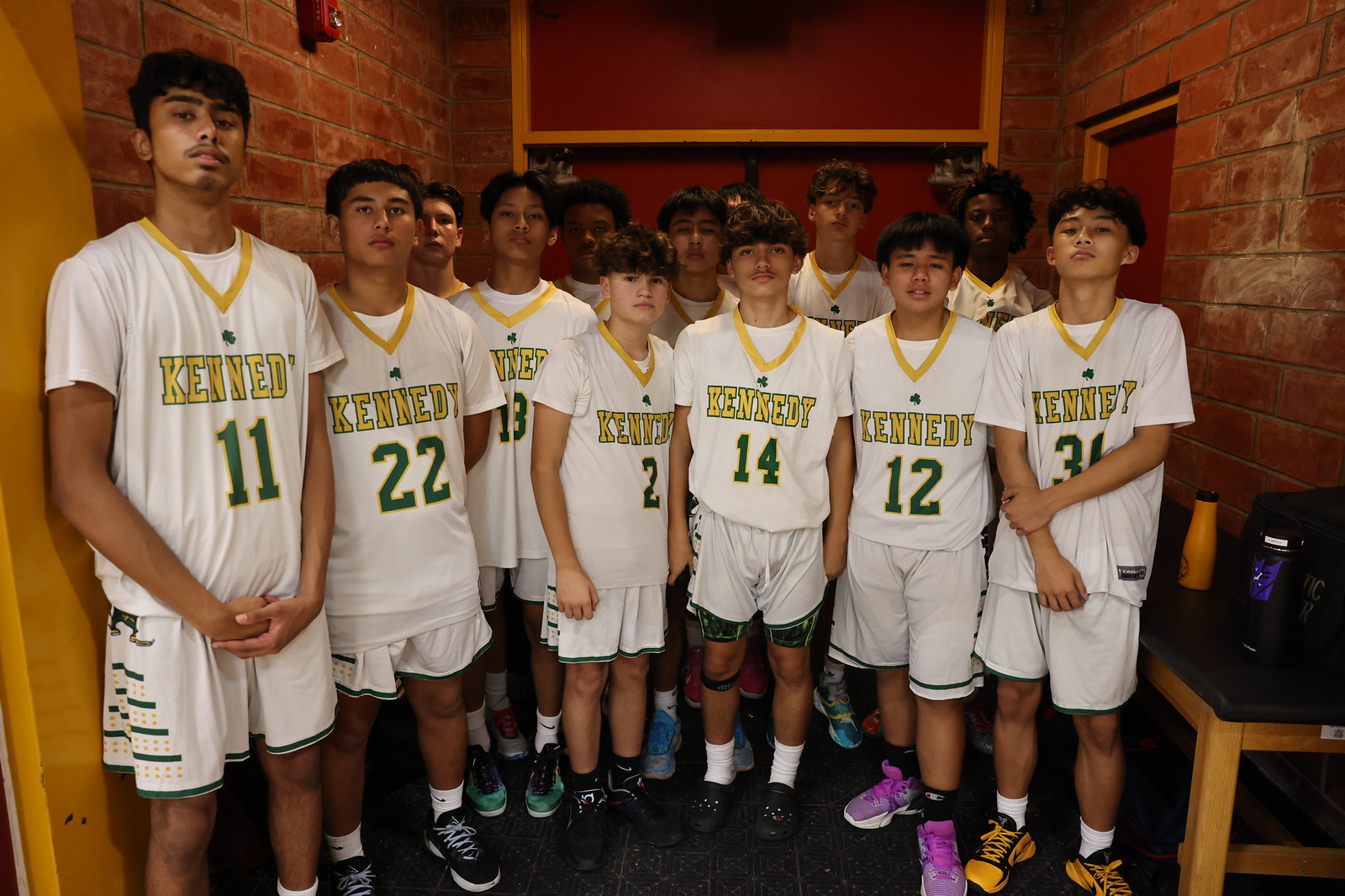The image captures a group photo of a boys' basketball team posing in a locker room. The team, predominantly composed of Hispanic members with tanned skin and a few black individuals at the back, is outfitted in matching uniforms. Each player wears a white jersey with "Kennedy" emblazoned in yellow letters, featuring a yellow V-neck trim, over a white undershirt, and paired with white shorts. The jerseys display various numbers: 11, 22, 13 or 18, 2, 14, 12, and 31. They sport a variety of basketball shoes, ranging in colors from black and white to more vibrant combinations like green, purple, and orange. The locker room setting is defined by red brick walls and an orange-framed door. In the upper left corner, a fire alarm is visible. On the right, a brown-legged bench with a blue top holds yellow and black bottles, alongside a dark-colored bag. The team stands closely together, posing eagerly for the camera.